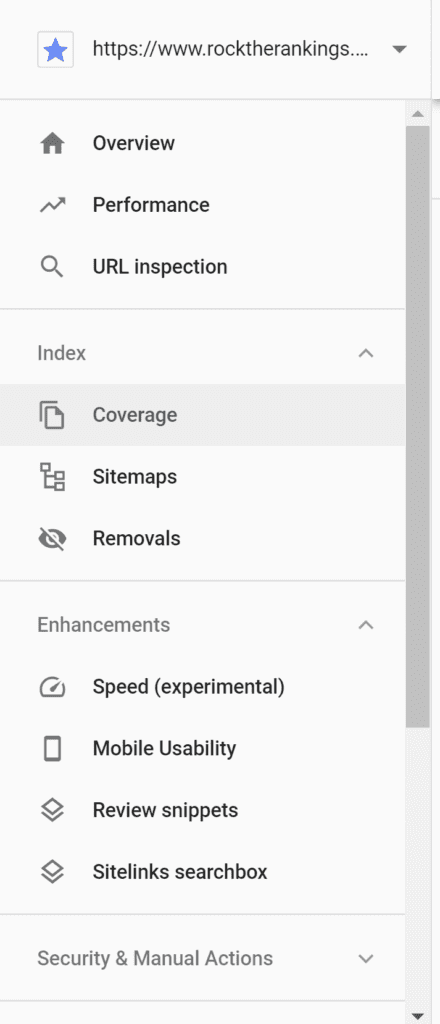Screenshot of a Smartphone Webpage

This image captures a screenshot taken from a smartphone, showcasing a web page with a predominantly white background. At the top, the web address is displayed as "https://www.rocktherankings" with a blue star icon to the left of the URL. Beneath the address, a gray line demarcates the boundary between the URL bar and the website's main content.

The main section of the webpage features various icons and titles, each representing different navigational options available on the site. These options include items such as "Overview," "Performance," "URL Inspection," "Coverage," "Sitemaps," "Removals," "Speed," "Mobile Usability," "Review Snippets," "Site Links," "Search Box," and "Security and Manual Actions." 

On the left-hand side of the screen, there is a scroll bar indicating that there are more items available than what is currently visible in the screenshot. The overall design appears clean and user-friendly, providing easy access to a range of tools and information for site management and analysis.